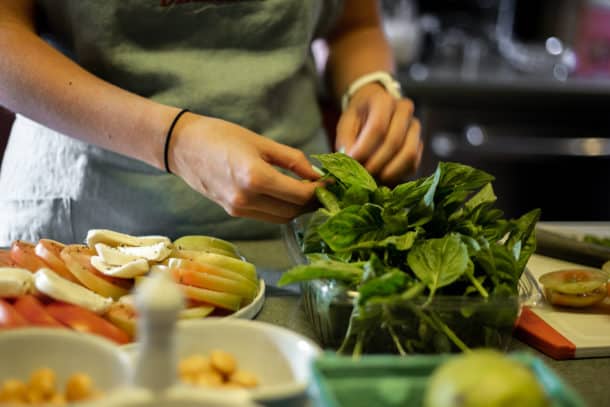In the image, there is a restaurant worker actively engaged in food preparation. The worker is wearing a snug, green apron that features a visible pocket. On their left wrist, they sport a white Apple Watch and a simple black band. The scene is set at what seems to be a buffet preparation station. The worker is handling fresh spinach with bare hands, notably without gloves, which is unusual for food handling. In front of them lies a tray laden with neatly sliced tomatoes and an assortment of other fruits presented on a platter. Adjacent to these items are several bowls containing various types of vegetables. To the right, a cutting block indicates ongoing preparation activities. In the background, although slightly blurred, either a stove or a series of cabinets and a kitchen sink can be seen, enhancing the busy kitchen environment. The overall scene suggests meticulous preparation for a buffet service.